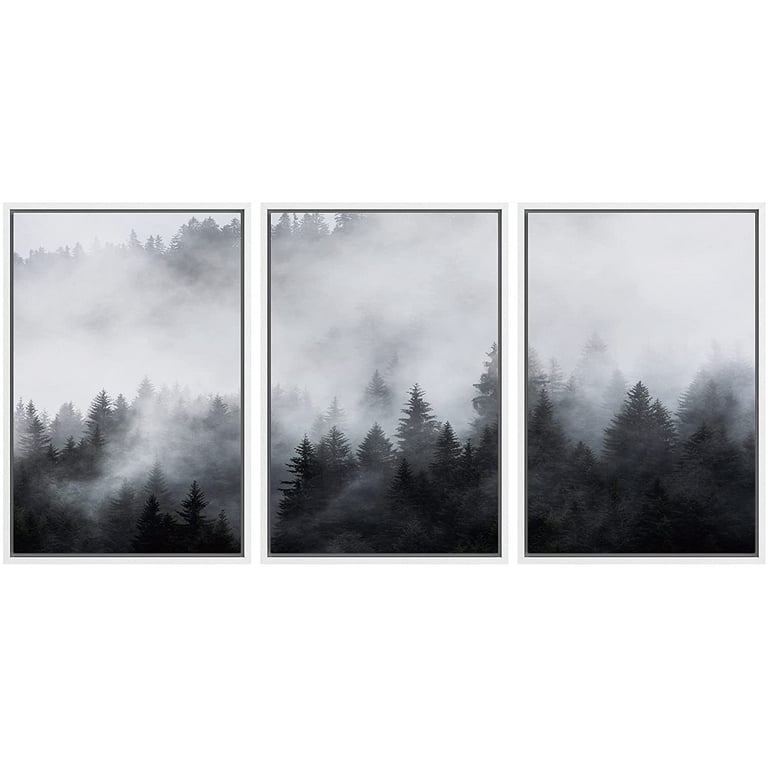The image displays a triptych of framed, black-and-white art photographs, each featuring a forest scene shrouded in mist. The three vertical rectangular photographs are bordered by thin white frames, accented with delicate black inner lines. The composition suggests that these images could align to form a continuous panorama, though small gaps between the frames interrupt the connection. 

Each photograph captures a different stage of a foggy forest landscape, likely observed from a hillside overlooking mist-filled valleys. The leftmost image shows shorter trees, with the fog thin enough to glimpse a skyline of distant tree tops and rocky bluffs. The middle image reveals a blend of shorter and taller trees engulfed in a thicker fog, predominantly concentrated on the right, while the left side is clearer. The rightmost photograph features the tallest trees, but the fog is so dense that the top half of the image fades almost entirely into white, obscuring any tree details. Together, these photographs create a dynamic visual narrative of a forest engulfed in varying densities of atmospheric fog.